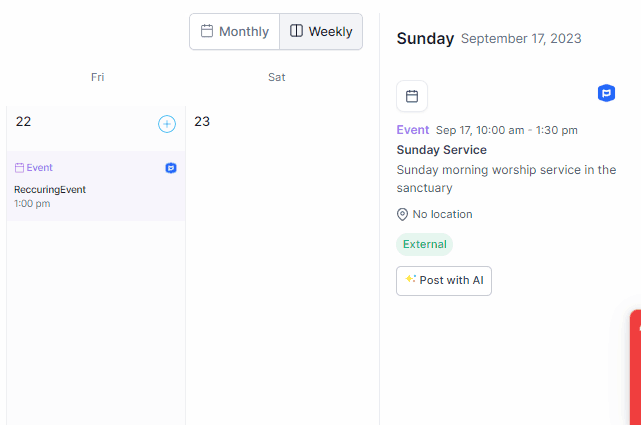Screenshot of a digital calendar displaying the 'Monthly' view for September. The visible dates include Friday, the 22nd and Saturday, the 23rd. There is a recurring event on Friday, September 22nd, at 1:00 p.m., simply titled "Recurring Event," with no additional details. On Sunday, September 17th, there's an event from 10:00 a.m. to 1:30 p.m. described as "Sunday Morning Worship Service in the Sanctuary." This event is marked as external with a green label, featuring a white button labeled "Post with AI," presumably to enhance or add further details to the event. The bottom right corner of the screenshot shows a cut-off red button, which might indicate an alert or notification.